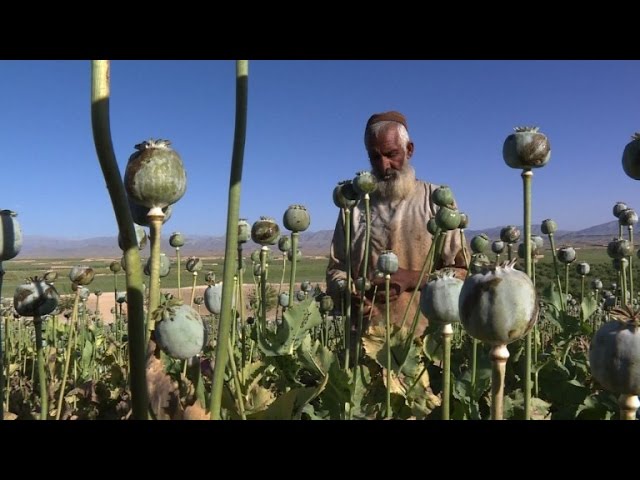The image depicts an older man with dark brown skin and white hair at the sides, transitioning to gray at the top, wearing a small brown hat. His attire consists of a light-colored, ragged shirt that darkens into brown towards the bottom, cinched with a dark brown waist belt. He stands in a sprawling field, surrounded by tall plants with spherical bulbs atop sturdy green stalks, resembling sunflowers or possibly poppies. The bulbs vary in color, some appearing whitish green and others dark green. The man appears partially obscured by the tall bulbs and foliage, which are the most sharply focused elements in the foreground. The background features another expansive field of similar plants, extending towards a backdrop of imposing mountain ranges under an unbroken, deep blue sky. The perspective of the image is low, almost at plant height, accentuating the vastness of the field and the serene yet rugged landscape. The image is bordered by black bars at the top and bottom, framing the scene from a distinct vantage point.